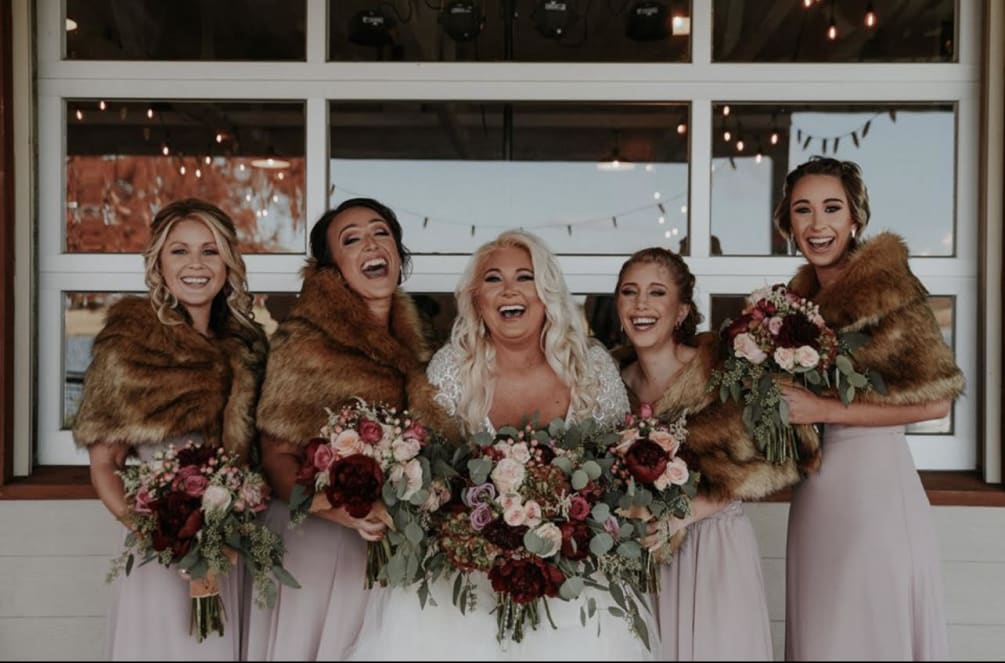In this photo, the joyful bridal party is centered around the smiling bride, who stands out in her elegant wedding dress with a short-sleeve lace bodice and a full white skirt. Her blonde hair complements her radiant expression as she holds an abundant bouquet featuring eucalyptus, white roses, pink and purple flowers. Flanking her are her four bridesmaids, each adorned in light pink dresses paired with brown fur stoles. Their similar bouquets echo the bride's floral arrangement. The group is positioned in front of a large garage door-style window, composed of glass panes, which reflects festooned lights suggesting an ongoing celebration outside. The backdrop is a simple white-painted concrete wall, enhancing the elegance of the scene.